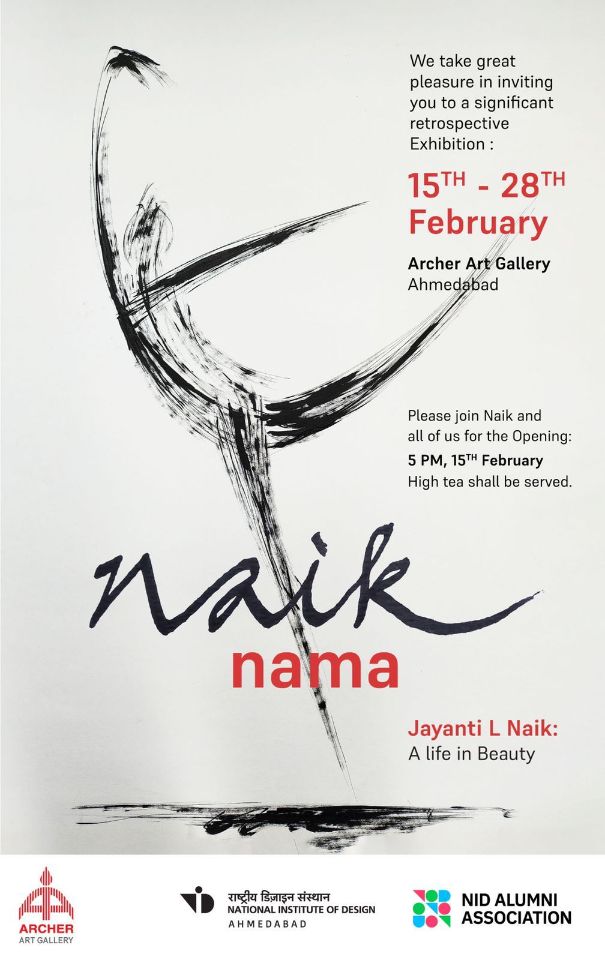This poster is an advertisement for a significant retrospective art exhibition titled "Jayanti L. Nayik: A Life in Beauty," taking place from the 15th to the 28th of February at the Archer Art Gallery in Ahmedabad. The central image consists of simple, abstract brush strokes that artfully depict a ballerina poised in mid-dance, balanced elegantly on one toe with her other leg extended behind her, one arm raised upward, and the other gracefully to her side, capturing the fluidity and grace of movement. 

Prominent text at the top of the poster reads, "We take great pleasure in inviting you to a significant retrospective exhibition," alongside details of the event's duration and venue. The opening reception is slated for 5 p.m. on the 15th of February, with an invitation to join Naik and others, and a note that high tea will be served. The name "Nayik Nama" is displayed prominently in the middle of the poster.

At the bottom of the poster, logos and names of sponsors and associated organizations are listed, including the Archer Art Gallery, National Institute of Design (NID), and NID Alumni Association.